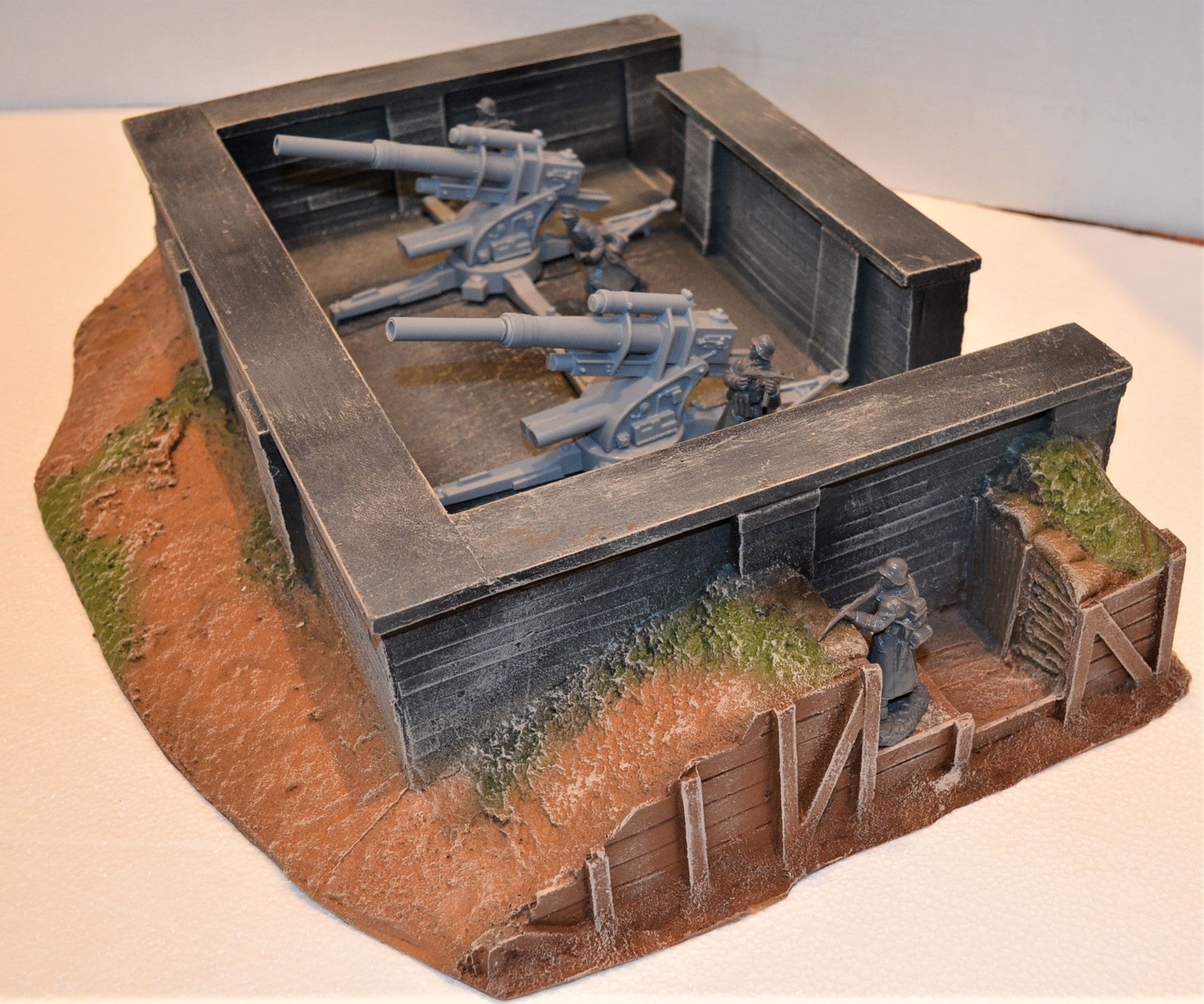This image depicts a detailed miniature model of a World War I or II fort. The fort is constructed with thick, dark brown barricades forming a shallow square, semi-protected from view. Inside the fort, two large, gray artillery pieces, possibly six-inch guns, are stationed behind the barricades. Three soldier figurines appear in the scene: two are positioned behind the artillery pieces inside the fort, while the third stands outside the fort in the dirt or sand, aiming a rifle. The surface of the model simulates a hill made of reddish-brown dirt with patches of green vegetation. There is also a wooden fence on the right side of the model. The setup rests on a white surface, highlighting the realistic and detailed craftsmanship of the miniature display.